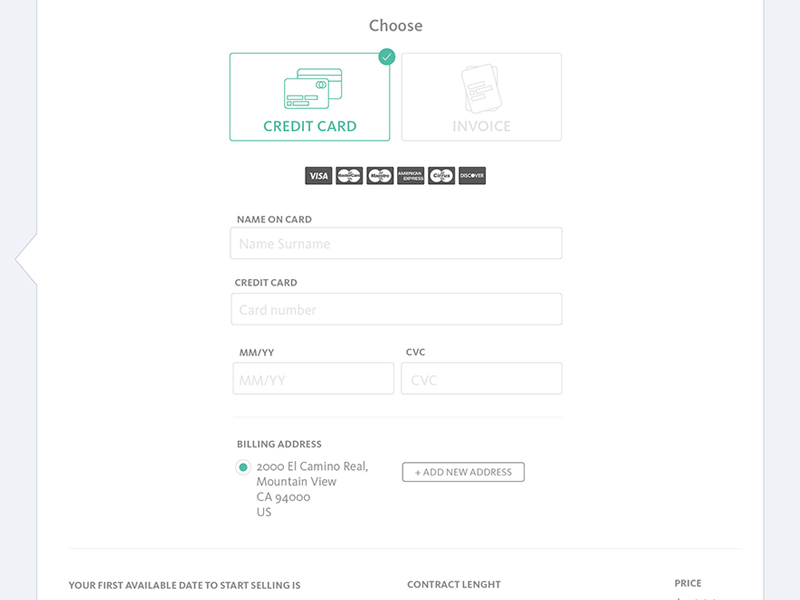The image depicts a payment interface. At the top, there is a section labeled "Choose." On the left side, the option "Credit Card" is highlighted in green, indicating it has been selected. On the right, the option "Invoice" is shown in grey. Both options are set against a white background.

The "Credit Card" section includes an illustration of a credit card outlined in green. Beneath it, there is a row of credit card logos, which includes Visa, two MasterCards, American Express, Discover, and another unidentified card.

Following that, there are fields for entering credit card information. The first field is labeled "Name on Card," with a sub-field labeled "Surname." Below, there are fields for entering the "Credit Card Number" with placeholder text in grey, "MM/YY" for the expiration date, and "CVC" for the card's security code.

A grey line separates the payment information from the billing address section below. Here, an address is pre-filled and selected: "2000 El Camino Real, Mountain View, California 94000, US." Next to this, a white button with a grey outline and text, marked with a plus sign, allows the addition of a new address.

At the bottom of the section, details regarding "Your first available date to start selling," "Contract Length," and "Price" are displayed.